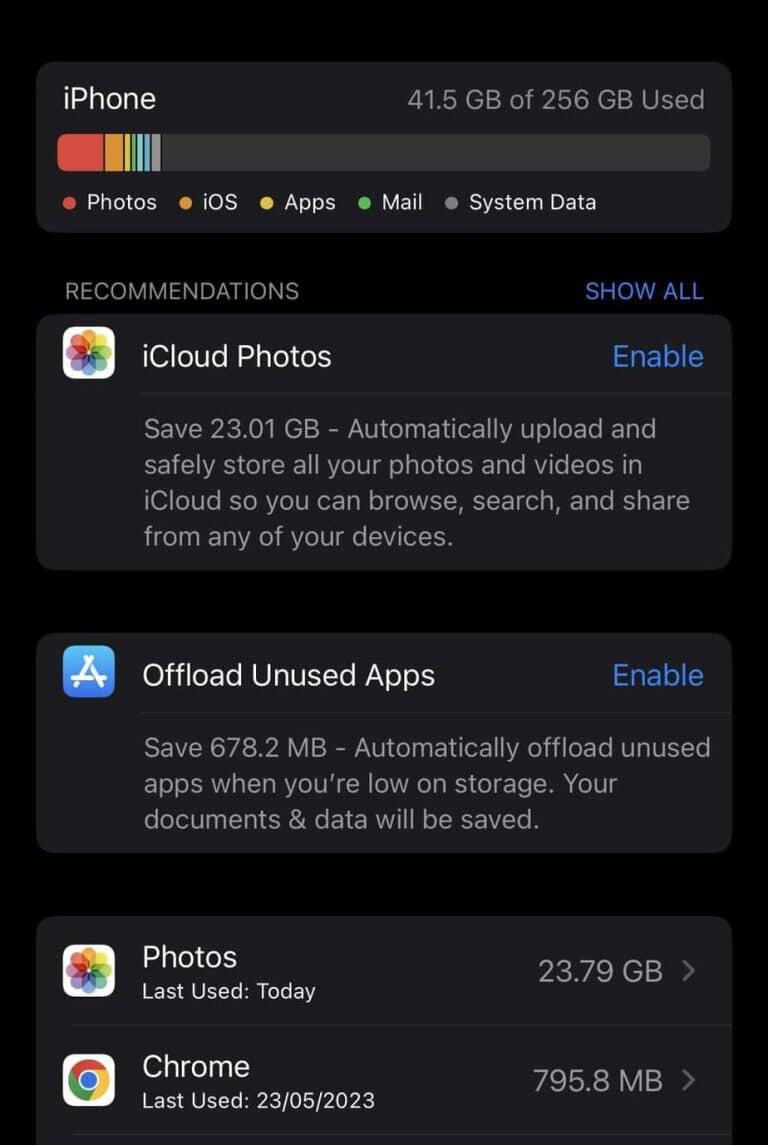This is an image of a smartphone displaying the storage settings screen. The background is predominantly black with four distinct sections in a lighter shade of black, arranged in a vertical list. At the very top, the word "iPhone" is prominently displayed, indicating the device in use. Beneath it, a storage bar graph shows that 41.5 GB out of a total 256 GB are used, with categorized sections marked in various colors. Categories such as Photos, iOS, Apps, Mail, and System Data are represented with small colored segments above the storage bar.

Below the storage usage summary is a section titled "Recommendations," featuring three suggestion boxes. The first box, labeled "iCloud Photos," has the familiar multicolored photo icon. The second box, "Offload Unused Apps," is identified with a blue icon featuring a white "A" in the center. The third box, which is partially cut off and labeled "Photos and Chrome," displays the Google Chrome logo, a multicolored circle. Each recommendation box includes an actionable option on the right side, with the top two suggesting activation buttons while the bottom box provides information about the amount of storage space used by the items listed.

The visual representation suggests that the phone has ample storage space remaining, with only a fraction of the total capacity utilized.